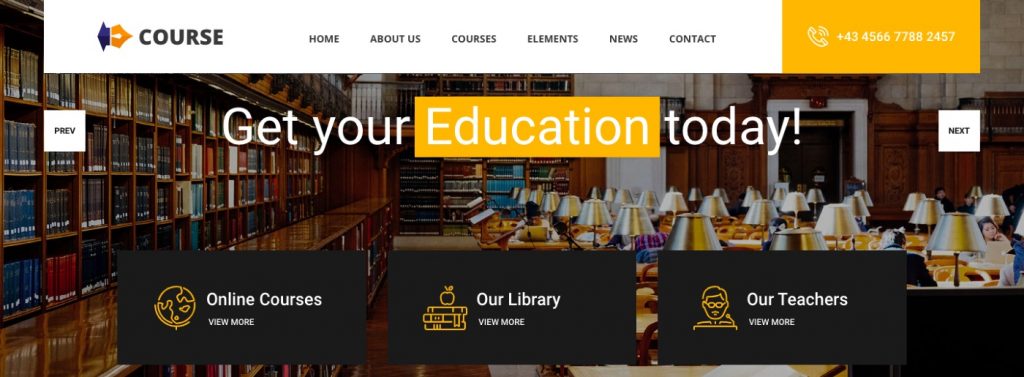The image depicts the home screen of a website for a company named "Course." The top left corner features the company's logo, which resembles a graduation tassel in shades of green, purple, and gold, positioned alongside the word "COURSE" in capital letters. 

The main navigation menu is rendered in uppercase black letters, listing the categories: HOME, ABOUT US, COURSES, ELEMENTS, NEWS, and CONTACT. To the right of the CONTACT tab is a yellow rectangular box containing both a phone and a sound icon, along with the phone number "+43-4566-7788-2457."

Beneath the navigation menu, on the left side, there's a box labeled "PREV." The title in the center of the screen reads "Get Your Education Today!" with the word "education" highlighted in a yellow box, followed by an exclamation mark. To the right of this title is another box labeled "NEXT."

Below the title, three subcategories are presented in black rectangular boxes, each accompanied by relevant icons: "Online Courses" with a globe icon, "Our Library" with a stack of books icon, and "Our Teachers" with a teacher icon. Each box includes a "View More" button.

The background of the entire scene is a photograph of a library, adding an educational ambiance to the website's home screen.